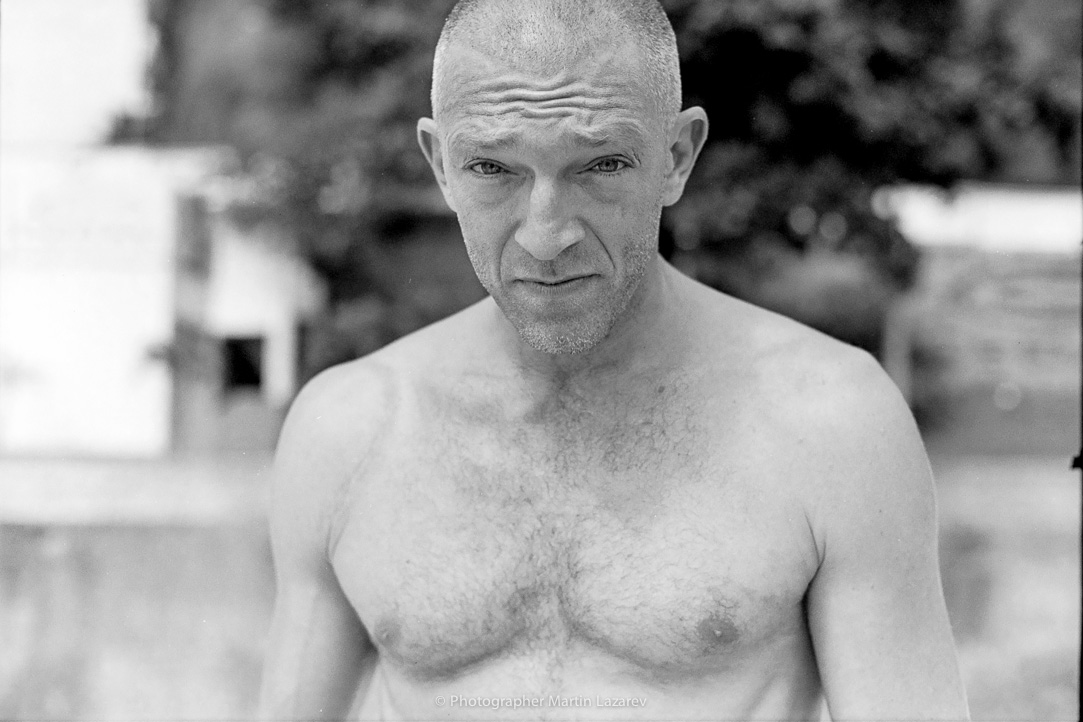The black and white photograph, taken by Photographer Martin Lazarev, captures a melancholic shirtless man with a buzz cut and a short beard, revealing a bit of stubble on his chin and sparse hair on his chest. Slightly slouched with his shoulders slumped, his lean physique hints at defined abs. His forehead is furrowed with pronounced wrinkles, and his eyes gaze upwards towards the camera, imparting a sad yet contemplative expression. The background is an indistinct blur, likely featuring large trees and potentially some buildings, consistent with an outdoor setting. Among the subtle tones of the image, the almost invisible white font at the bottom discreetly credits the photographer.